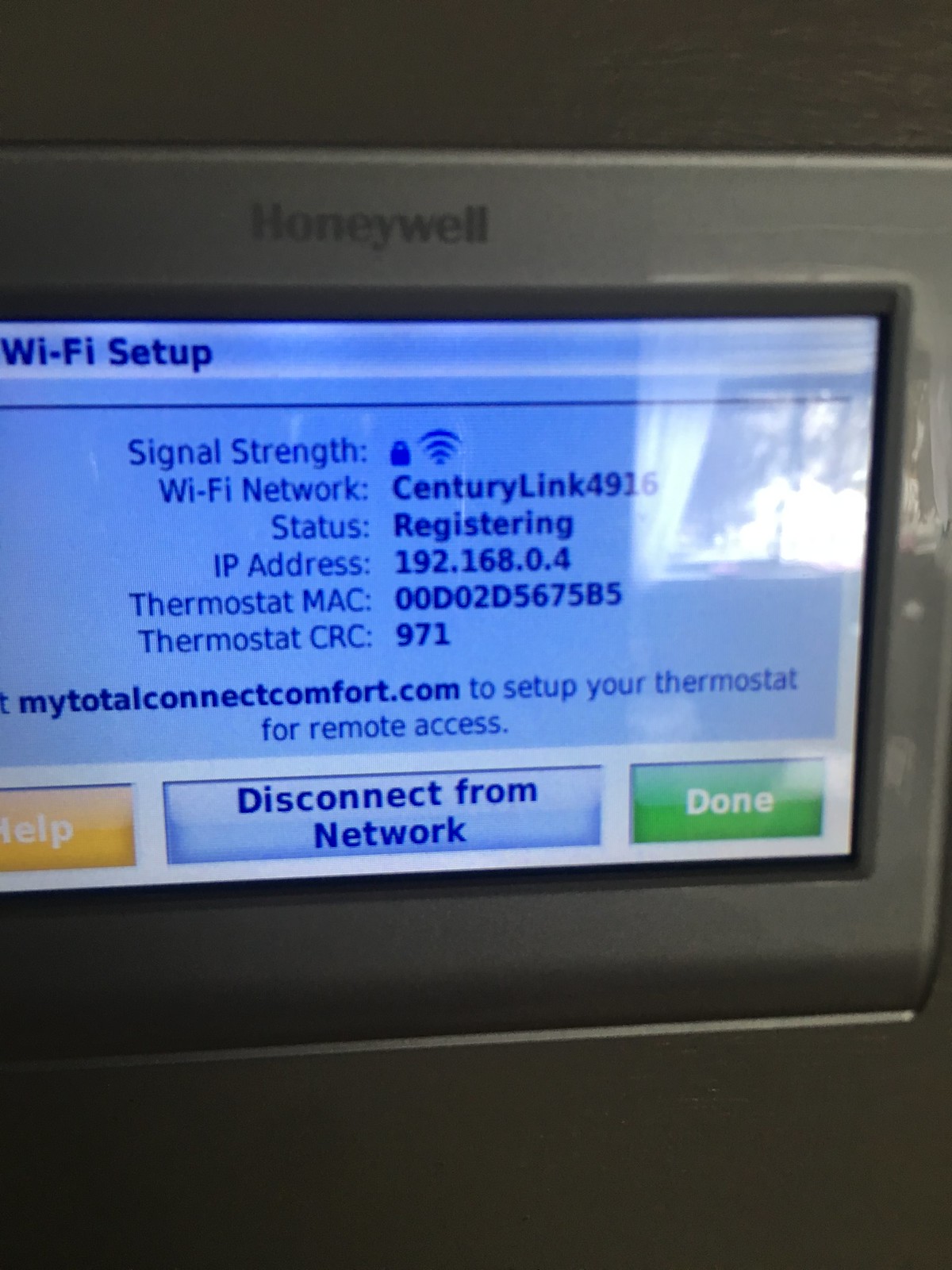The image showcases a Honeywell thermostat with a light blue glass screen prominently displaying its Wi-Fi setup interface. At the top of the device, the brand name "Honeywell" is clearly visible. The screen is organized with detailed information about the Wi-Fi connection. Notably, it lists the Wi-Fi network as "CenturyLynx 4916" and the signal strength. The status indicates "registry," and the IP address is displayed as "192.168.0.4." Additional details on the screen include the thermostat MAC address "00:D0:2D:56:75:B5" and the thermostat CRC "971." Situated at the bottom of the screen are three colored buttons: a yellow "Help" button, a blue "Disconnect from Network" button, and a green "Done" button, providing users with various options to manage the Wi-Fi configuration.